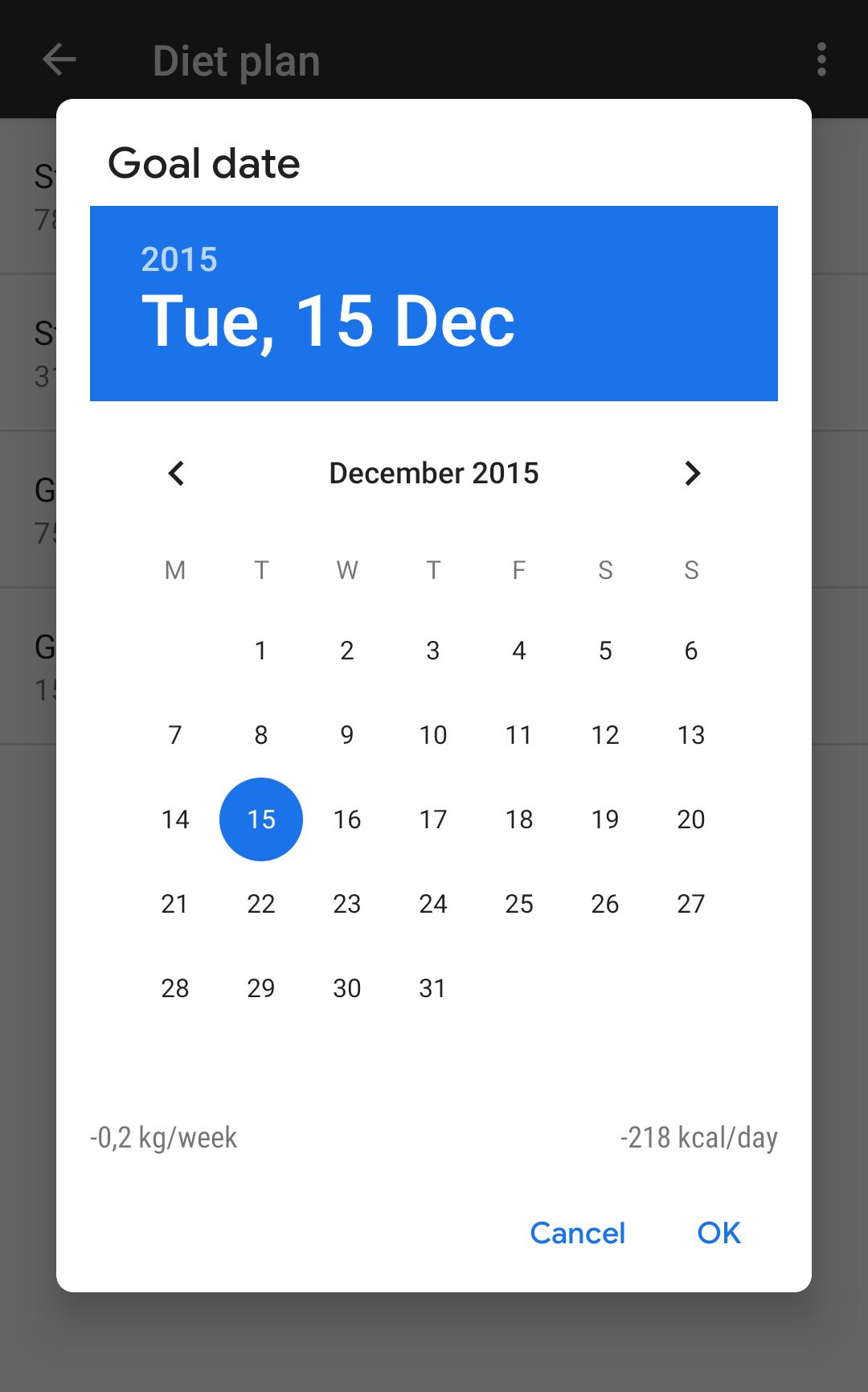A detailed view of a diet plan calendar is obstructed by a pop-up window with a white background and rounded edges. The pop-up, titled "Gold Date," features a prominent blue stripe at the top displaying "2015, Tuesday, 15th December" in white text. Immediately below the stripe is the December 2015 calendar. Notably, this particular month comprises 31 days, beginning on a Tuesday and concluding on a Thursday. In the bottom left corner of the pop-up, there is text indicating "2kg week, negative, 0, 2kg week," and to its right, it reads "negative 218 kcal a day." At the bottom right corner of the popup, there are clickable links or buttons labeled "Cancel" and "OK." The partially obscured diet plan calendar remains visible behind the pop-up window.